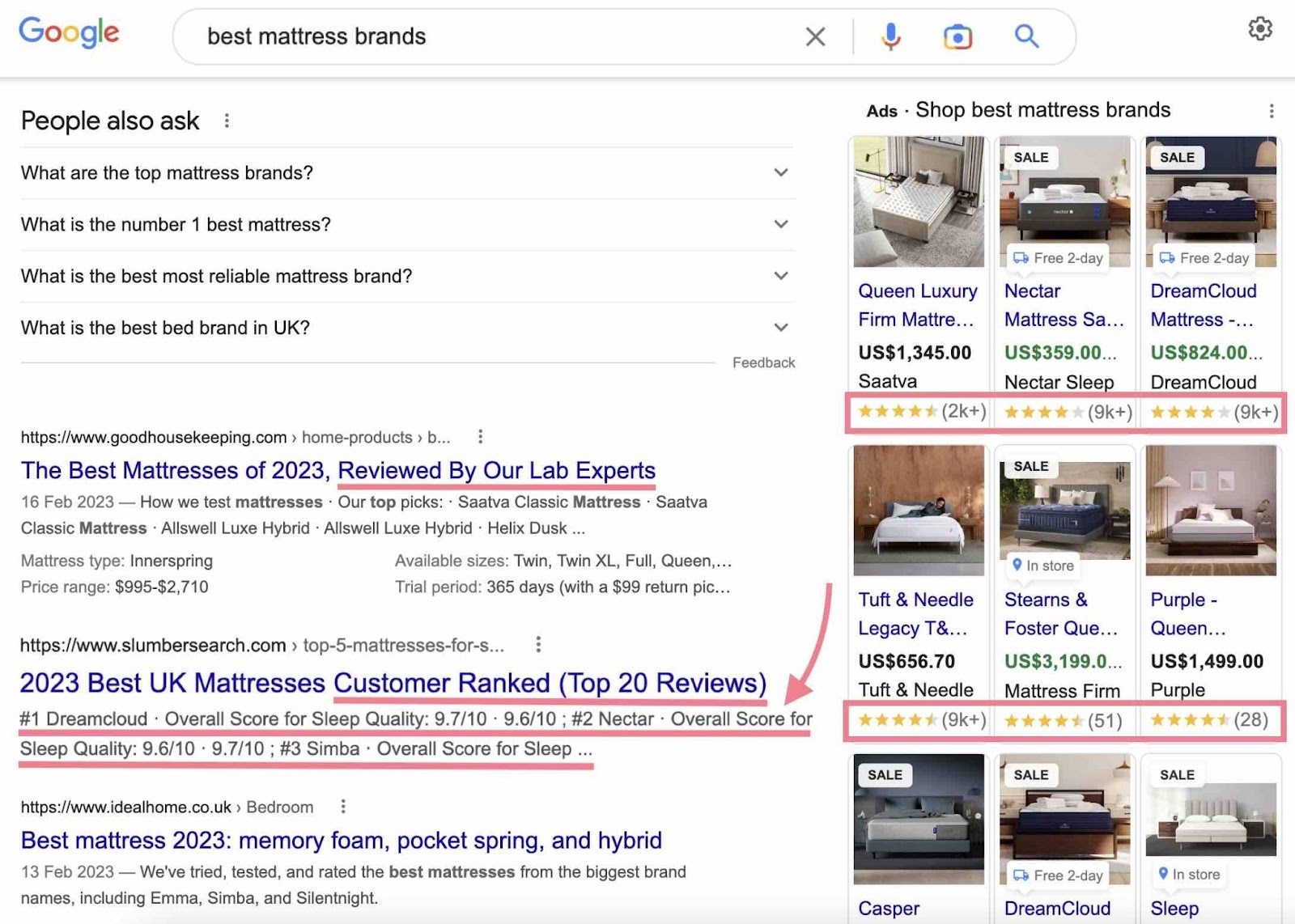This Google search page displays a query for "best mattress brands" at the top. The Google logo is positioned in the upper left corner, showcasing the iconic colors of red, gold, blue, and green. Below the search bar, which includes an 'X', a microphone icon, a camera icon, and a search icon, there are several suggested search queries such as "What are the top mattress brands?", "What is the number one mattress?", "Best mattress", "What is the best most reliable mattress brand?", and "What is the best bed brand in the UK?"

Among the search results, the first highlighted entry reads, "The best mattress of 2023 reviewed by our expert lab." The text is underlined in red. The next result features "2023 best UK mattresses" alongside a customer-ranked list of the top 20 reviews, also underlined in red. An eye-catching pink arrow directs attention to the customer-ranked reviews.

Further down, another result is titled "Best mattresses 2023: Memory foam, pocket spring, and hybrid." On the right side of the page, a section labeled "Shop best mattress brands" displays various mattress brands and their prices, allowing for easy comparison before making a purchase.